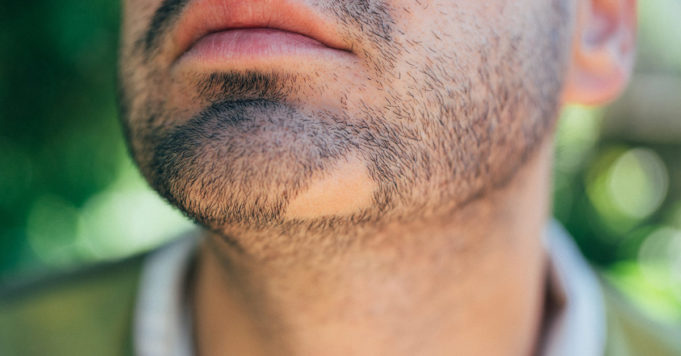This image presents an extreme close-up of a man's face, focusing from his upper lip to the midsection of his neck. He has several days' growth of a dark beard, distinguished by a small, triangular patch of bare skin on the left side of his chin where no hair grows at all. His skin is light tan. The background is a blur of green shades, likely suggesting foliage, indicating the photograph might have been taken outside. His attire includes a green shirt with a white collar, although the shirt itself is partially blurred.